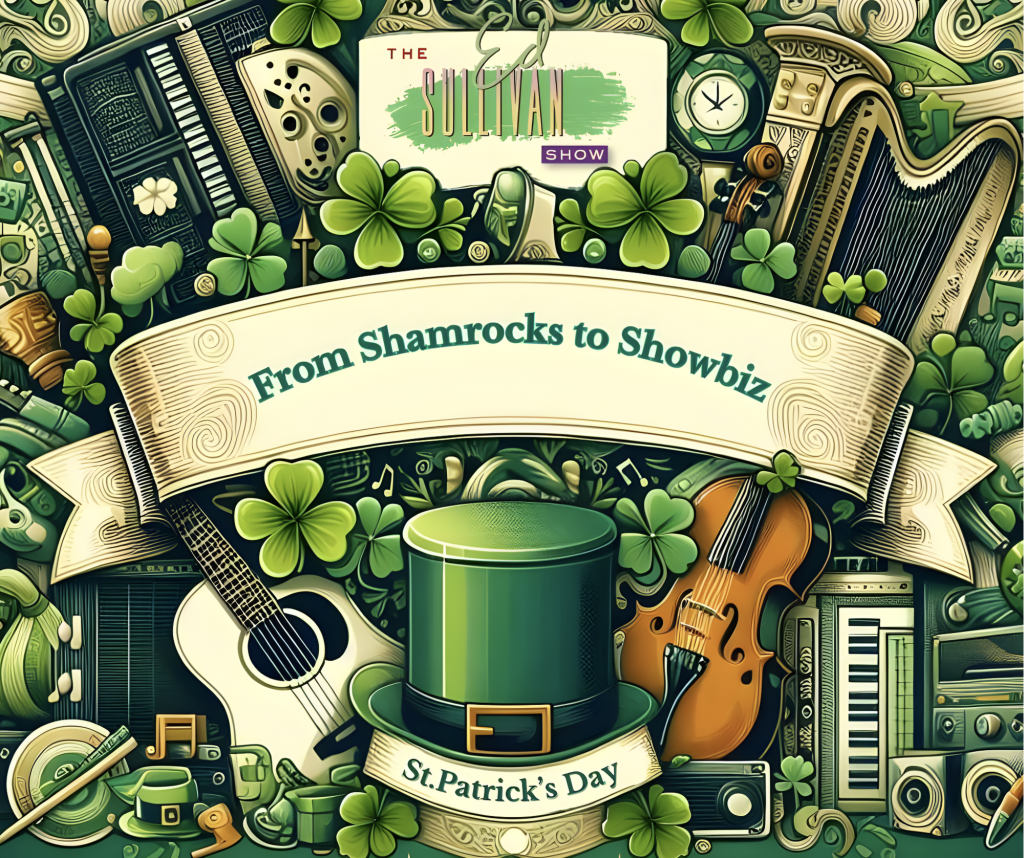This is a vibrant, complex graphic with a variety of cartoon and illustrator-style clip art elements. Dominating the top center of the image is a white box that reads "The Ed Sullivan Show," with "Sullivan" presented in a gradient from pink to yellow and set against a green paint splash. Above it, "Ed" is written in a cursive green font. 

Framing this central piece are numerous eclectic objects that often appear AI-generated due to their oddly blended details. Featured prominently is a clock with four hands, instruments like an unidentifiable keyboard adorned with a flower and string elements, a hybrid of a harp, trumpet, and violin, along with separate depictions of traditional instruments such as a guitar, acoustic guitar, orange violin, and possibly a flute and an accordion. 

A light gold banner across the middle declares "From Shamrocks to Showbiz" in green text, reinforcing the Irish theme with scattered shamrocks, clovers, and intricate gold and green filigree. Underneath, a green leprechaun hat sits above another banner proclaiming "St. Patrick's Day." Around these, additional items like another keyboard, speaker-like squares, a possible cassette player, music notes, and a yellow-green target with a stick add to the thematic clutter.

Despite the chaotic arrangement, the large banners and musical instruments stand out against the predominantly green and tan color scheme, embellished with splashes of gold. The overall style is highly jumbled, making it challenging to discern individual objects aside from the banners and major instrument motifs.